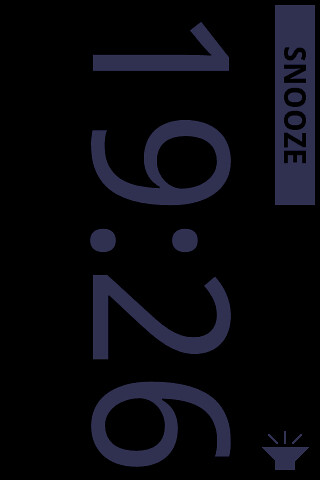This image is a digitally illustrated graphic with a black background. Dominating the image is the word "snooze" written in a dark blue-grey color, though it is rotated 90 degrees, requiring one to turn their head or the image itself to read it properly. Across the main part of the image, a 24-hour format digital time "19:26" is prominently displayed. Situated at the bottom is an icon resembling a torch, emitting three lines that symbolize light rays. The minimalist design bears a resemblance to interface illustrations commonly seen on mobile phone screens. There are no additional elements or decorations within the image.